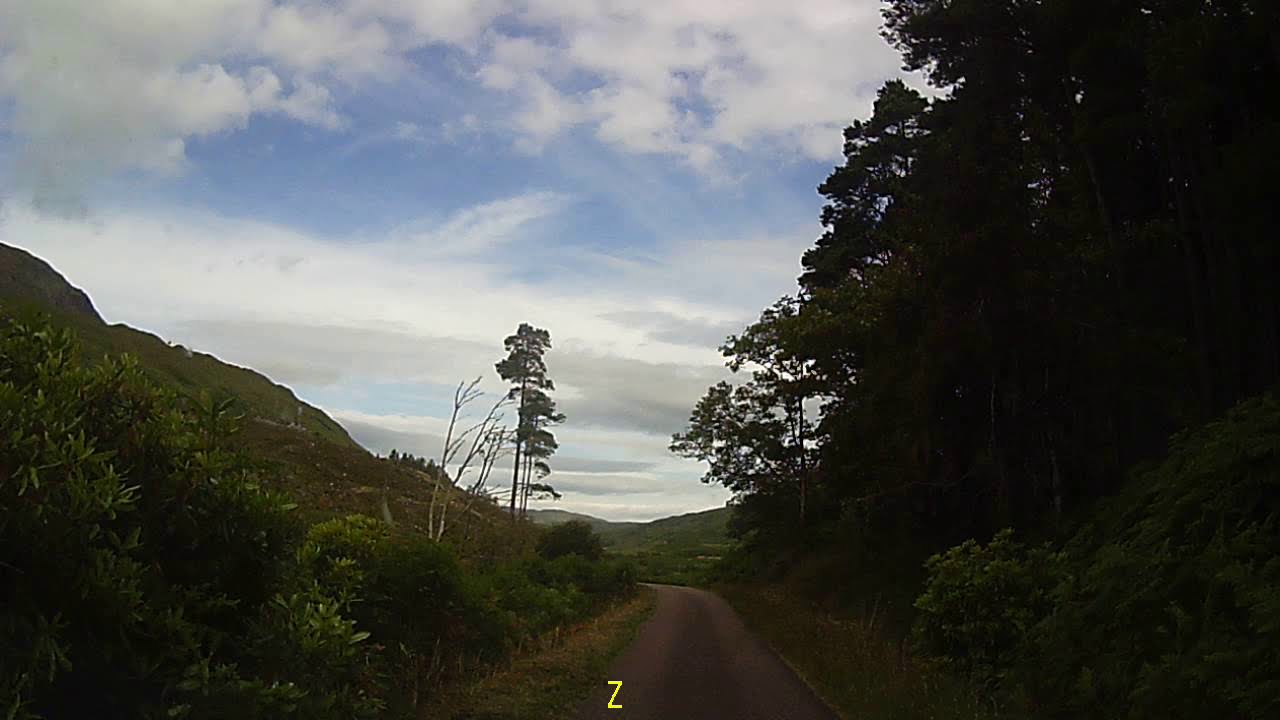The image captures a serene outdoor scene dominated by a winding dirt road that curves gently to the left before disappearing from view. The road is flanked by varying greenery on both sides, including tall green grass, shrubs, and trees with thin trunks. Some trees are fully leafed, while others are sparse or bare. To the left of the road, there is a low hill covered in bushes and shrubs, with a prominent tree in the foreground partially shrouded in shadow due to the foliage. To the right, a taller, hillier area is densely packed with green trees and shrubs. In the distance, more hills stretch across the horizon, adding depth to the landscape. The sky above is a light blue dotted with scattered gray and white clouds, creating a calm and somewhat cool atmosphere. The entire scene is cast in the soft shadow of the trees, giving it a dim yet tranquil ambiance. Notably, there is a yellow letter "Z" at the bottom of the image, possibly marking or annotating the photograph. The overall effect is one of a peaceful, secluded path in a lush, hilly terrain, far from any paved roads or urban hustle.